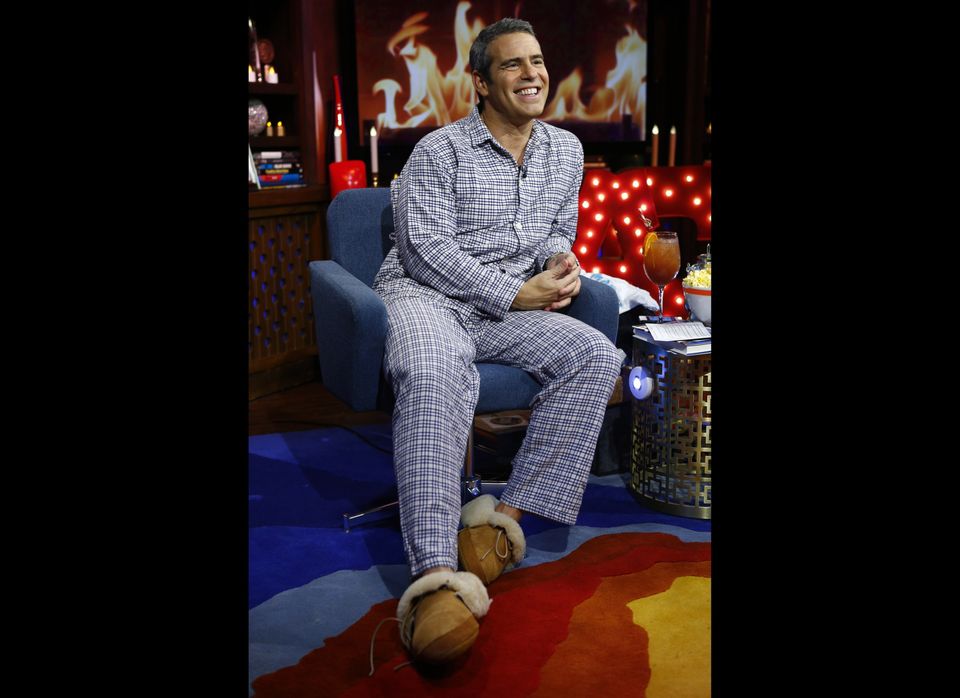In this detailed picture, we see a man, likely in his late 40s, sitting comfortably in a blue fabric chair with metal legs. He's dressed in a matching set of blue plaid pajamas, featuring a button-down shirt and long pants, complemented by brown furry moccasin-style indoor slippers. The man is smiling broadly and looking slightly upwards, his hands folded over his lap, exuding a relaxed and pleasant demeanor.

Next to him is a small side table on which rests a glass of what appears to be a murky brown drink, possibly wine, and a partially visible bowl of popcorn. There is also a book on the table. Behind the man is a vibrant area rug with lines of yellow, orange, red, light blue, and dark blue.

The scene is set against a backdrop of several lit candles and an electronic fireplace that adds a warm, cozy ambiance. Additionally, there are illuminated letters behind him, including a visible "A," contributing to the atmospheric lighting. A dark brown bookshelf with upper cabinets and lower shelves is seen in the upper left corner, framing the setting further. The overall setting presents a cozy and inviting environment, perfect for a relaxed evening at home.